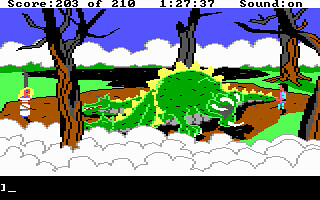The image captures a dynamic screenshot from a retro-styled arcade or video game. The sky forms a gradient from a deep blue at the top to white clouds clustered along the horizon. Below the sky, the landscape consists of green grass interspersed with barren, dead trees, their lifeless stumps and limbs scattered sporadically. Dominating the background, a large, enigmatic vat filled with an ominous black substance—possibly a deep hole or a lake of black liquid—adds to the scene's intrigue.

Prominently featured in the foreground is a billowing mass of white smoke, contrasting sharply against the vivid scenery. At the center, the focal point of the image, stands a formidable two-headed green dragon, its menacing presence hinting at an imminent battle or challenge. To the right, a character garbed in blue and sporting pink skin faces off against this beast, ready for action. On the left side, a distressed woman with blonde hair appears helplessly tied up, possibly implying a rescue mission.

Across the top of the image, a black font displays vital game statistics: a score of 203 out of a possible 210, a timestamp reading 1:27:37, and an indication that sound is on. Additionally, the scene is framed by a black bar at the bottom of the screen, likely reserved for in-game text or player instructions. This dense array of visual and textual elements paints a vivid picture of an intense and captivating moment within the game.